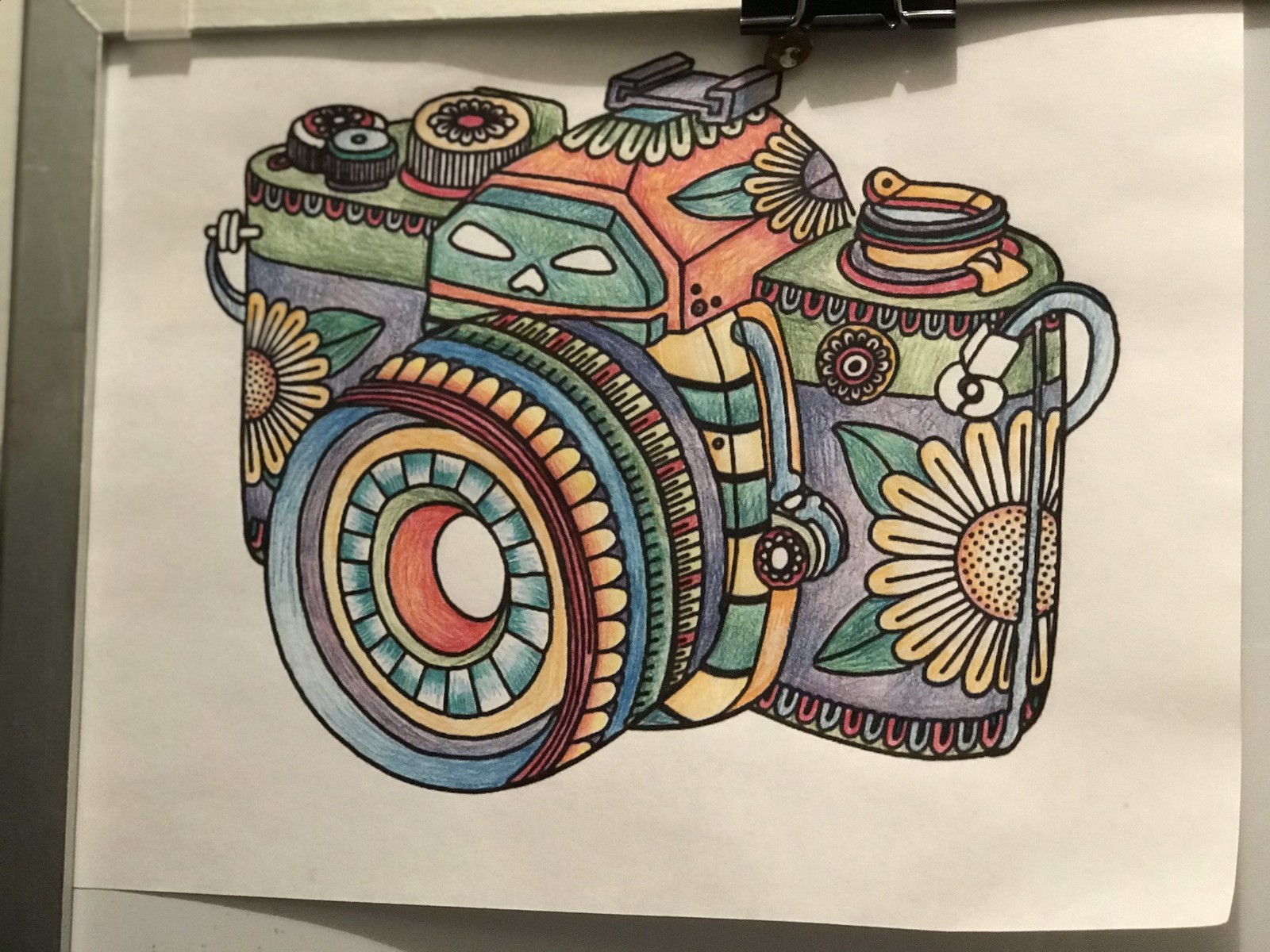A close-up photograph of a colorful, stylized drawing of a single-lens reflex camera is clamped to a piece of white paper on a white table. One black clamp is visible at the top of the image. The camera, painted in a vibrant, watercolor-like style, incorporates various bold colors including blue, purple, yellow, green, red, and orange. The main body of the camera is decorated with yellow sunflowers that have orange centers and dark green leaves. The lens, which appears kaleidoscopic and cylindrical, features an intricate pattern with hues of yellow, purple, dark blue, orange, olive green, cyan, and teal. Detailed designs such as white eyes and a nose on a green face are seen where the trapezoidal flash mount would be. The top buttons are adorned with multicolored patterns and floral designs, and the top of the camera is painted green.